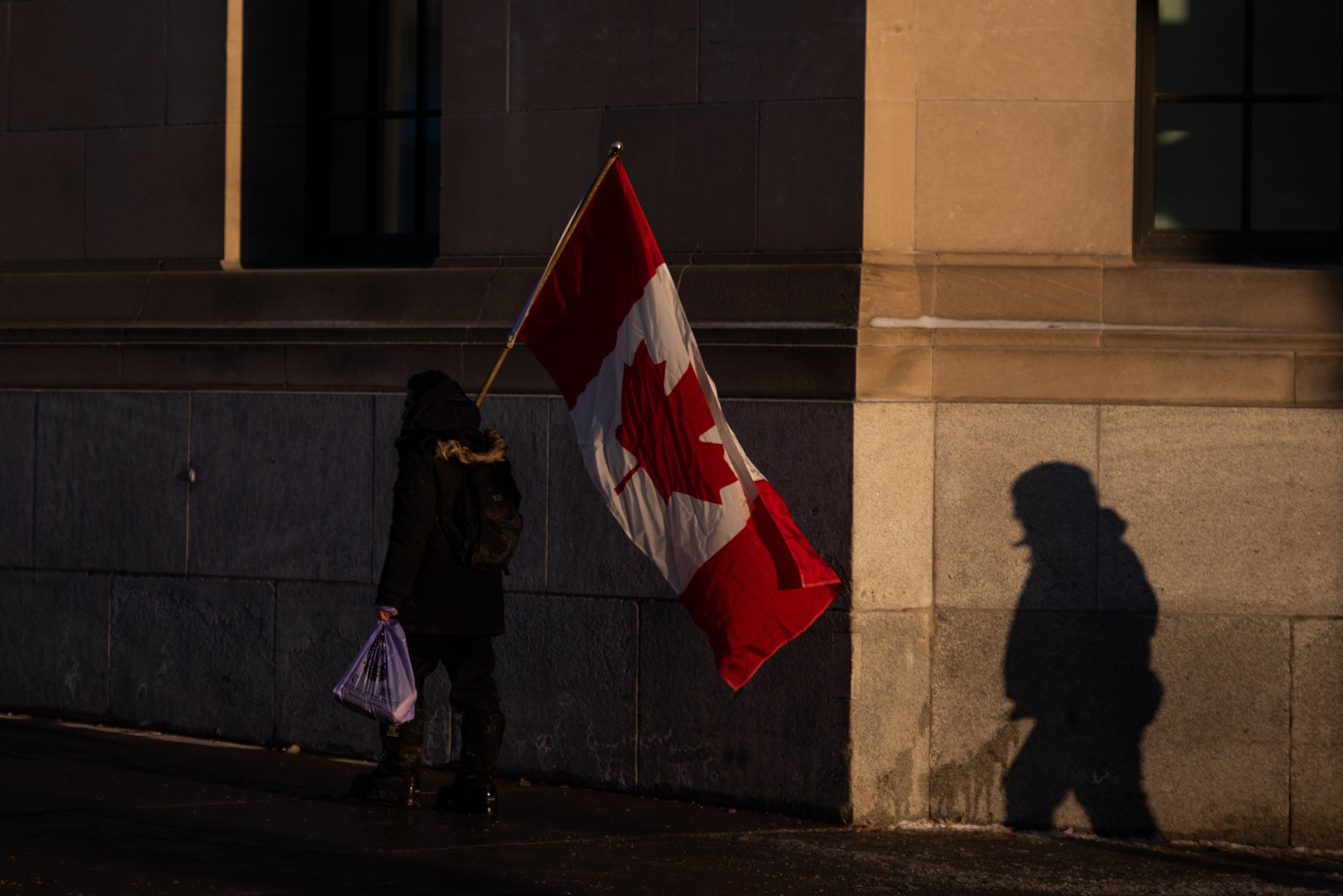The photograph depicts a solitary pedestrian walking uphill on a dimly lit city street, either at dawn or nighttime. The scene captures the person, dressed entirely in dark clothing including black boots, pants, jacket, backpack, and a fur-lined hood, as they move from the bottom right to the upper left of the image. They carry a gray or purplish plastic bag in their left hand and a wooden pole with a Canadian flag—characterized by its iconic red and white stripes with a central red maple leaf—in their right hand. The person is positioned between the left and central thirds of the photo, walking adjacent to a brick and cement building. This building has large, black-framed windows at head level and gray cement stones at the foundation, transitioning to mostly brown and tan stones as they ascend. Additionally, on the right side of the corner, the shadow of another person, partially visible, appears on the wall, hinting at their imminent entrance into the frame.